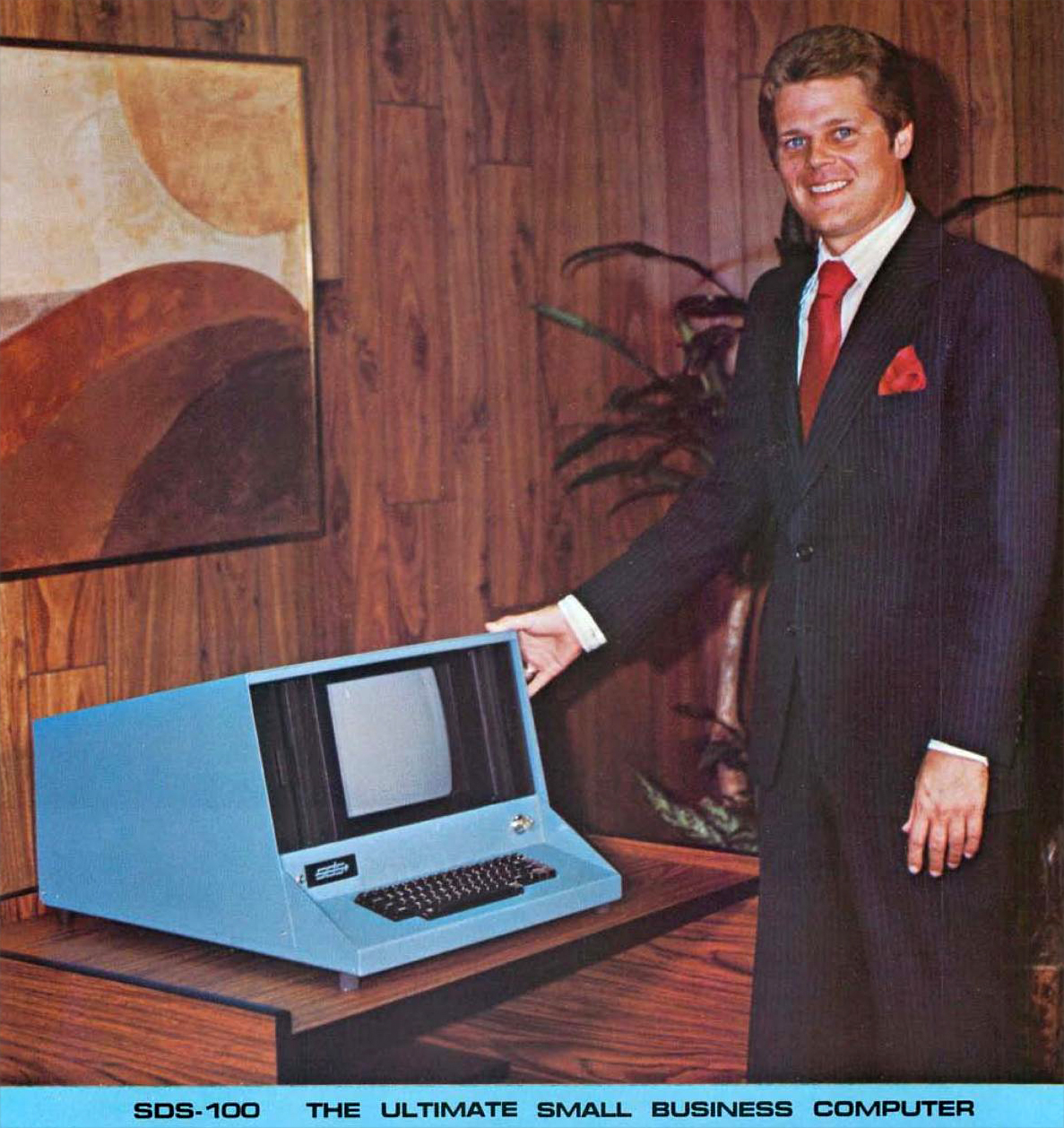The image showcases a vintage scene, likely from the early 1980s, set in a wood-paneled room. In the center, a gentleman with short blonde hair and blue eyes stands smiling in front of an old, boxy blue computer labeled "SDS-100: The ultimate small business computer." The man is dressed in a dark blue pinstripe suit with a white shirt, a red tie, and a red handkerchief in his coat pocket. The computer, an all-in-one model featuring a small screen with a black frame and an integrated black keyboard, is positioned on a wood-grain laminate desk. Just above the computer, a painting adorns the wall, depicting a yellowish sky, a brown ground, and a sun in the corner. The nostalgic atmosphere is highlighted by the period-specific details, including the wood paneling and the "ultimate small business computer" marking on the machine, emphasizing the early computing era.